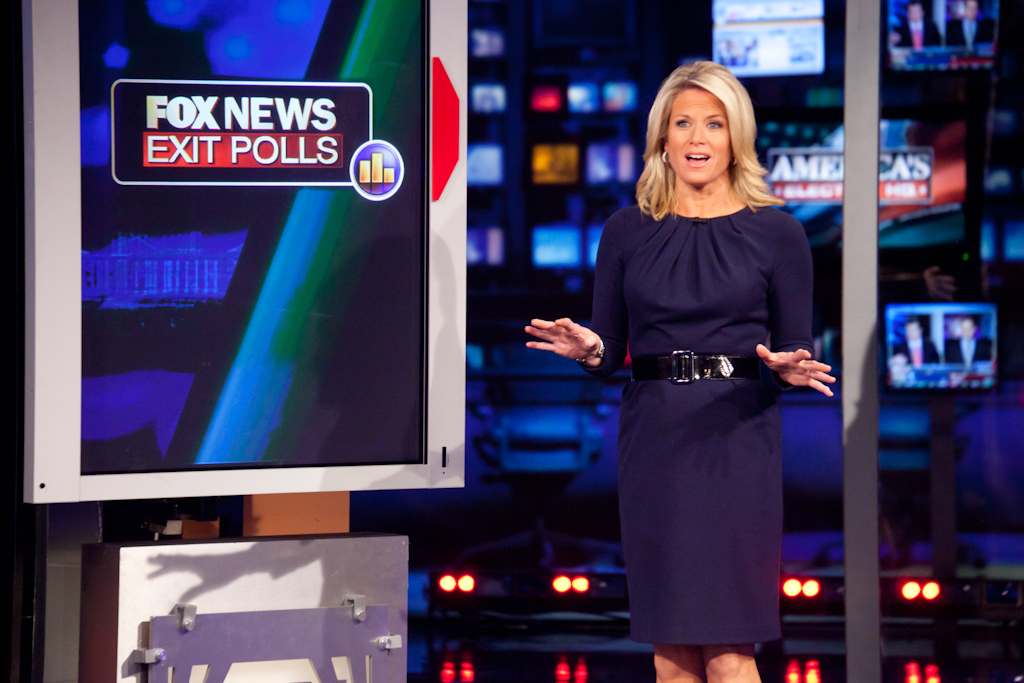In this TV screenshot, a blonde-haired news reporter with shoulder-length hair is broadcasting on Fox News, discussing exit polls. She’s dressed in a vibrant blue, long-sleeved dress that reaches just above her knees and is cinched at the waist with a black belt. Her hands are outstretched mid-discussion, and she wears noticeable earrings. Behind her, the studio background is slightly out of focus, featuring an assortment of monitors. Prominently among them is a screen labeled "Fox News Exit Polls" in white text, set against a detailed graphic that includes a combination of Tetris-like pieces in red. Additionally, several screens display two men in black jackets, likely part of the news team, repeated in the upper right corner.